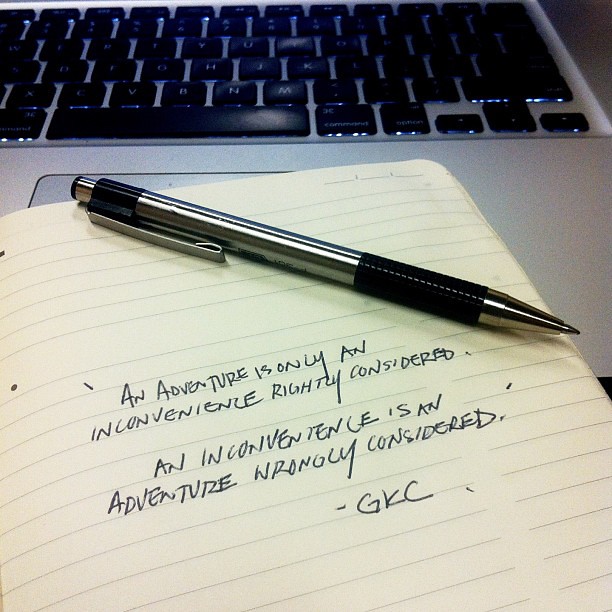The photograph appears to be designed as a stock image, featuring a neatly arranged scene that includes a white-yellow ruled paper notebook and a laptop. The open notebook, positioned slightly askew, reveals a single page with a handwritten quote in black ink: "An adventure is only an inconvenience rightly considered. An inconvenience is an adventure wrongly considered. - GKC." This phrase is written using a silver pen with a black grip, which rests horizontally across the top of the page. The notebook lies partially over the touchpad area of the laptop, allowing the laptop's silver frame and black keyboard to be visible in the background, giving the impression that the workspace is ready for use. The setup, though simplistic, is intentional and evocative of a moment paused for reflection or inspiration.